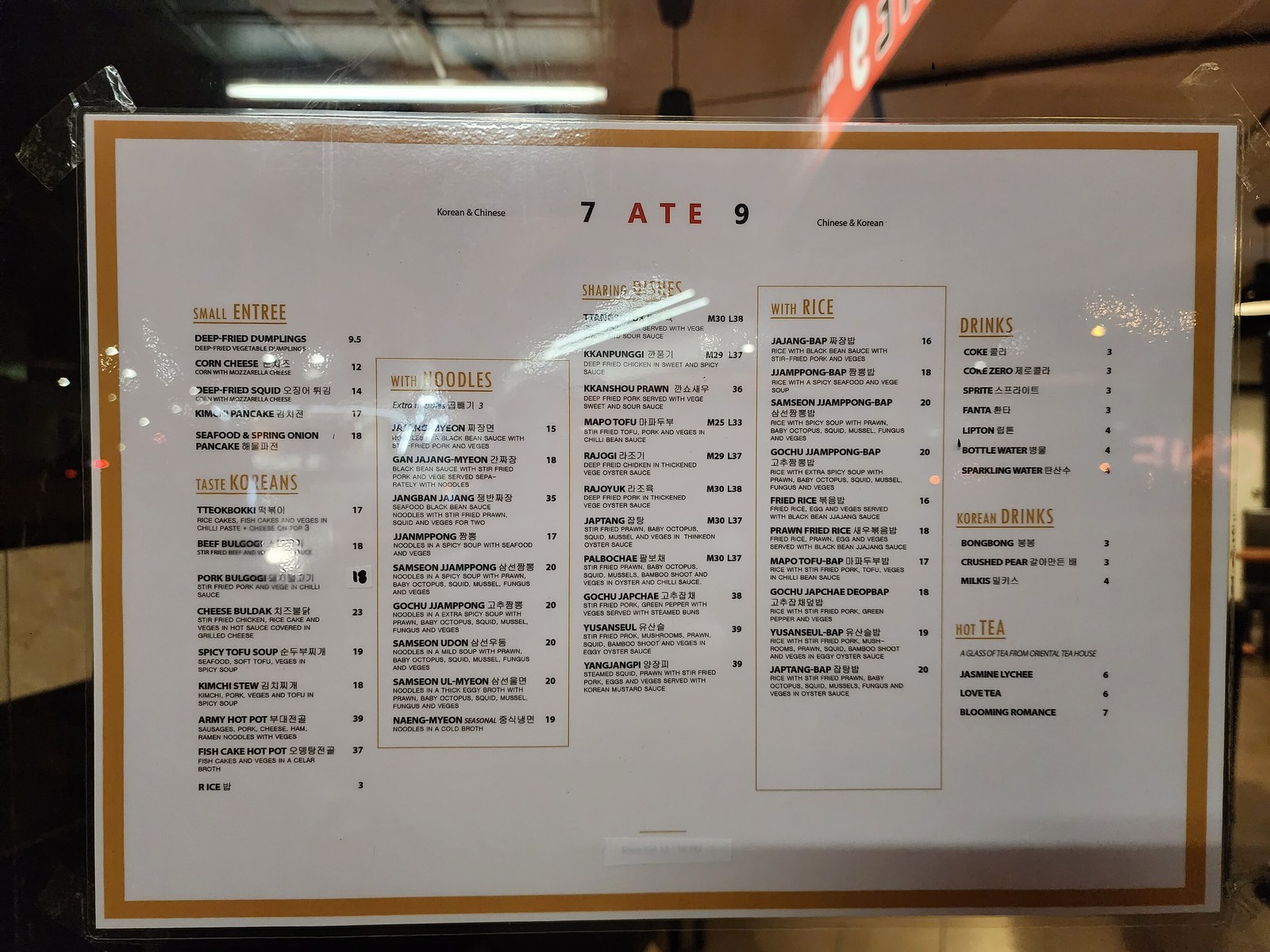This close-up photograph captures a plastic menu taped to a window, each corner secured with clear scotch tape. The menu features a white background and is adorned with an orange border at the top, where "789" is prominently displayed. The "8" stands out as it is stylized with the word "A-T-E" in red letters, while the "7" and "9" are in black. On either side of "789," small black text is printed, although it's not legible in the photo. 

The primary focus of the menu is the detailed list of dishes and their prices, organized into categories. The category names, such as "Small Entree," are indicated in orange font. Under this particular category, the text "Taste Koreans" is visible on the left side. Other categories are also present but not detailed in this description.

Through the window, the interior of the restaurant is subtly visible. The background features a large, hanging fluorescent light fixture at the very top and a portion of a ceiling fan in the center, hinting at the ambiance within.